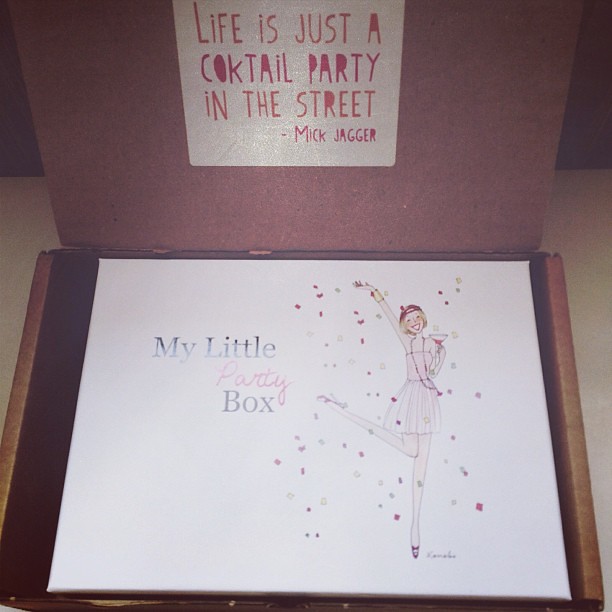The image showcases a brown cardboard box with its lid open and propped up. On the lid, in a playful festive font with pink and dark purple lettering, a quote from Mick Jagger reads, "Life is just a cocktail party in the street." The letters feature artistic embellishments, with the circles in letters like A, O, P, and R filled in with various colors. Inside the box rests a smaller, white box against a pink background. This smaller box is adorned with the label "My Little Party Box" to the left in black print, with "Party" highlighted in pink cursive. Beside the label on the right side, a hand-drawn image of a lively woman with blonde hair in a light pink dress is featured. She is holding a glass of wine in her left hand, with her right hand raised, as she balances gracefully on her left leg. Surrounding her, a vivid cascade of confetti in shades of purple, white, pink, and yellow adds to the celebratory mood. The photograph, cropped into a square, captures a light tan tabletop as the backdrop for this festive setup.